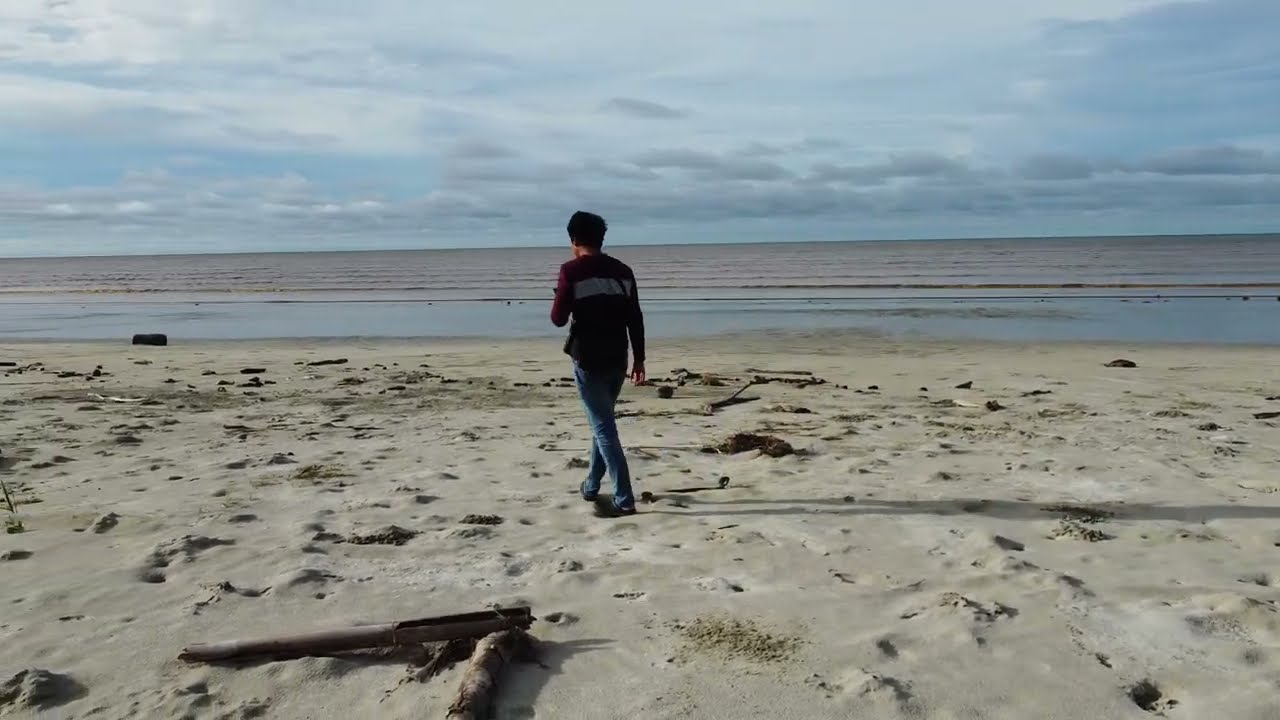In this image, we are on a damp, sandy beach, possibly after a rain or at low tide. A man with short dark hair is seen from behind, walking towards the calm, brownish ocean water. He is wearing blue jeans and a dark sweatshirt that has a purple hue with a gray stripe across the middle. The beach is scattered with pieces of driftwood and small mounds of sand, among which patches of green weeds are visible. The water is smooth with gentle, low waves caressing the shoreline. The sky overhead is mostly overcast, filled with dark clouds, although hints of blue sky peek through. The overall scene captures a tranquil, slightly gloomy day at the beach.